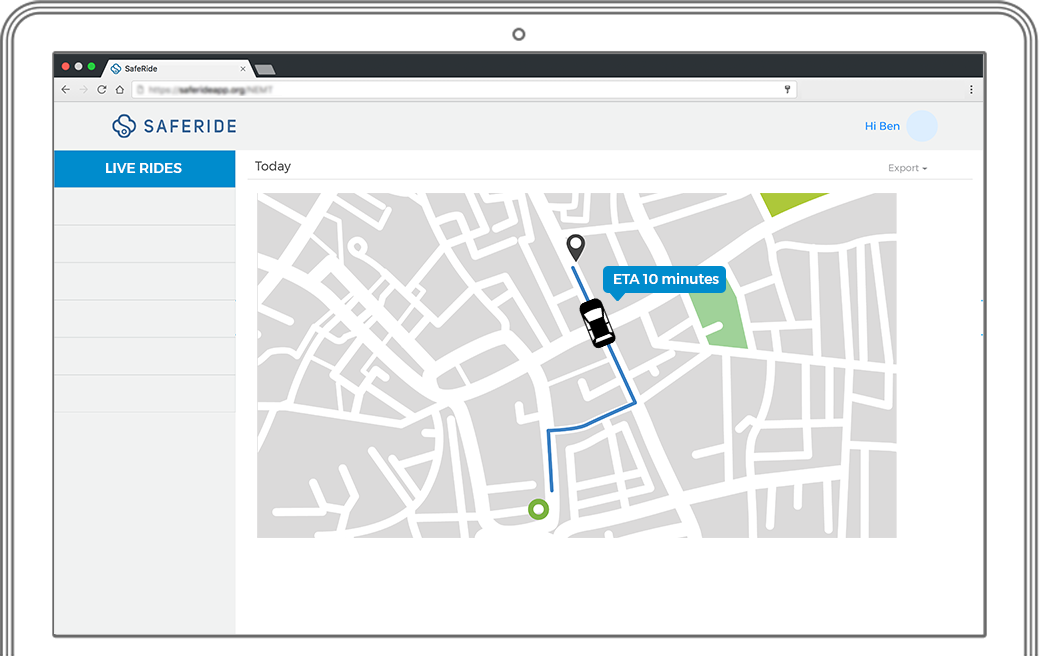This detailed screen capture showcases a computer monitor embedded within a digital mock-up, adding a gray frame to the image mimicking an actual monitor. The focus of the display is a browser window featuring the SafeRide website. On the left side of the webpage is the SafeRide logo, a small blue emblem accompanied by the business name "SafeRide" in text. Directly below this, a vertical navigation menu is prominently visible, with the "Live Rides" tab selected in blue. The main content area of the page is dominated by a large, stylized map, rendering a simplified street layout in gray with white streets. Covering a segment of this map is a blue line indicating a route. Centrally located within this route is a black car icon, accompanied by a call-out bubble displaying the message "ETA 10 minutes," providing a real-time update on the car’s estimated time of arrival.